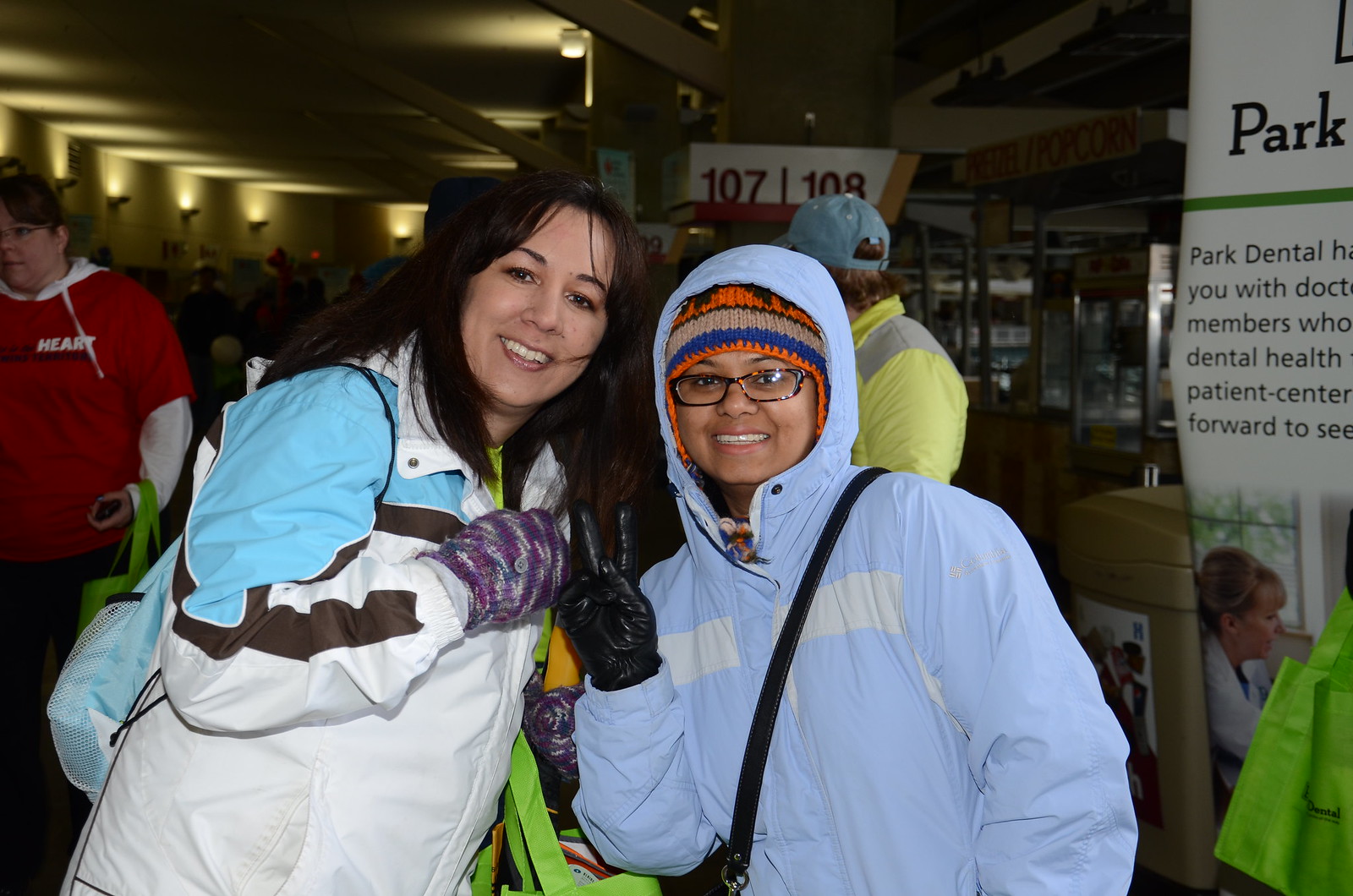In this image, we see two women posing for the camera, smiling warmly. Both are dressed in winter attire, suggesting a cold environment. The woman on the left has long straight brown hair and is wearing a white jacket with blue shoulders and a brown stripe. She has on purple mittens and she’s leaning toward the other woman. The woman on the right is wearing a very light blue winter jacket with the hood pulled over her head and a multicolored beanie in black, orange, brown, and blue. She also has black gloves and is making a peace sign with her right hand, while her glasses are visible under the beanie. Both have tote bags, possibly filled with swag, slung over their shoulders. In the background, there is a partial sign reading "Park Dental," hinting that this might be a convention, possibly a dental convention. The scene is set indoors with lighting sconces illuminating the long hallway, adding to the sense of a bustling interior space.